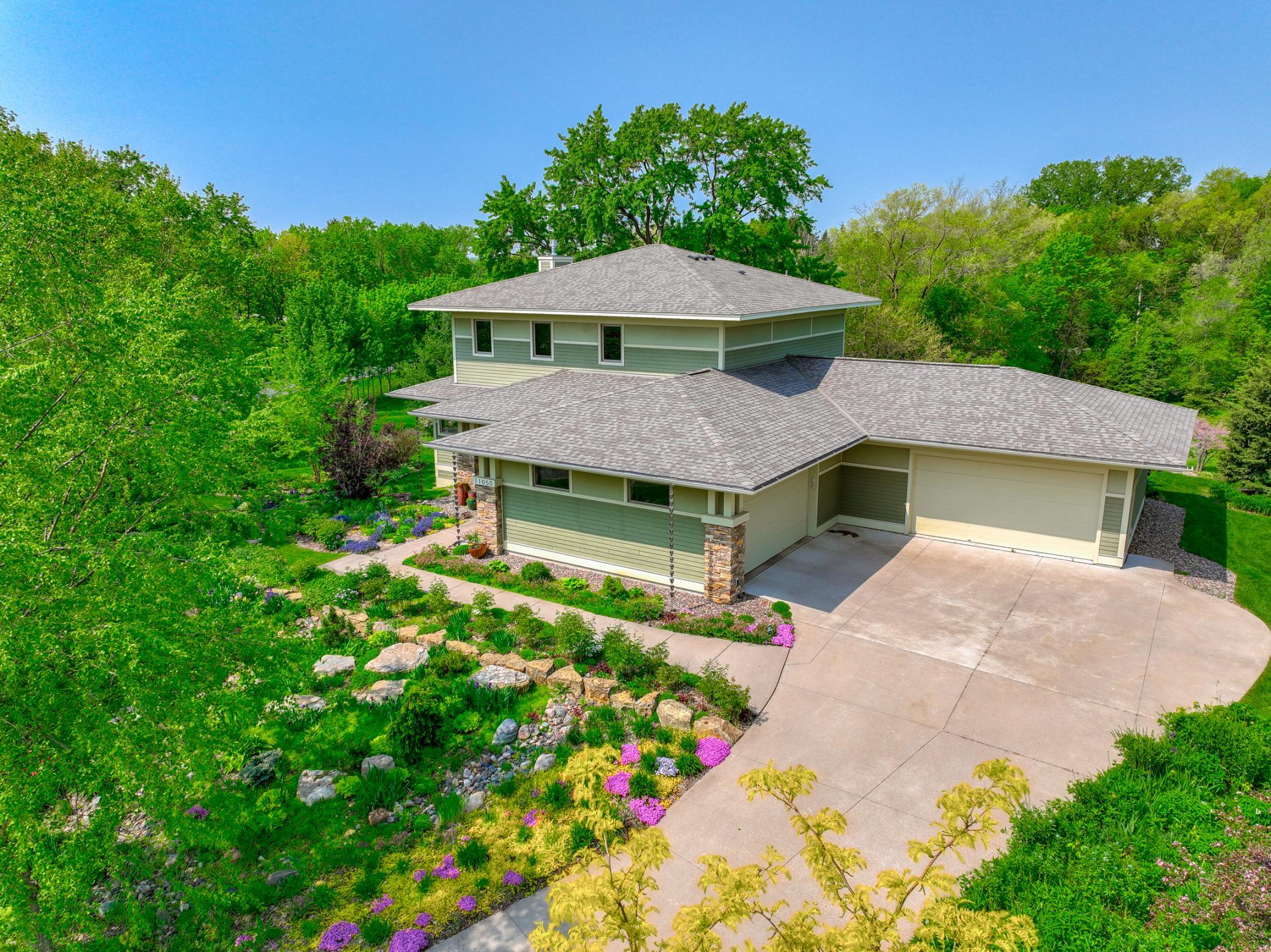This photograph, likely taken from a drone, captures a picturesque rural two-story house surrounded by an abundance of greenery and trees. The house features a blend of green shades, with light green siding on the top, followed by a row of darker green and then very light green beneath. It has a brown-tiled roof and three black-framed windows on the upper floor. The garage door, positioned centrally at the bottom, is light green with a white strip across the base flanked by columns made of orange-colored rocks. 

The driveway, composed of a mixture of light gray and orange concrete, is situated on the right side. A concrete sidewalk leads from the driveway to the front door. The vibrant garden includes flowerbeds with purple, yellow, and blue flowers and a tree with light yellow leaves situated prominently in the front yard. Beyond the house, large green trees give an impression of a lush, park-like setting, with no other dwellings in sight, emphasizing the serene and secluded nature of this beautiful rural property.